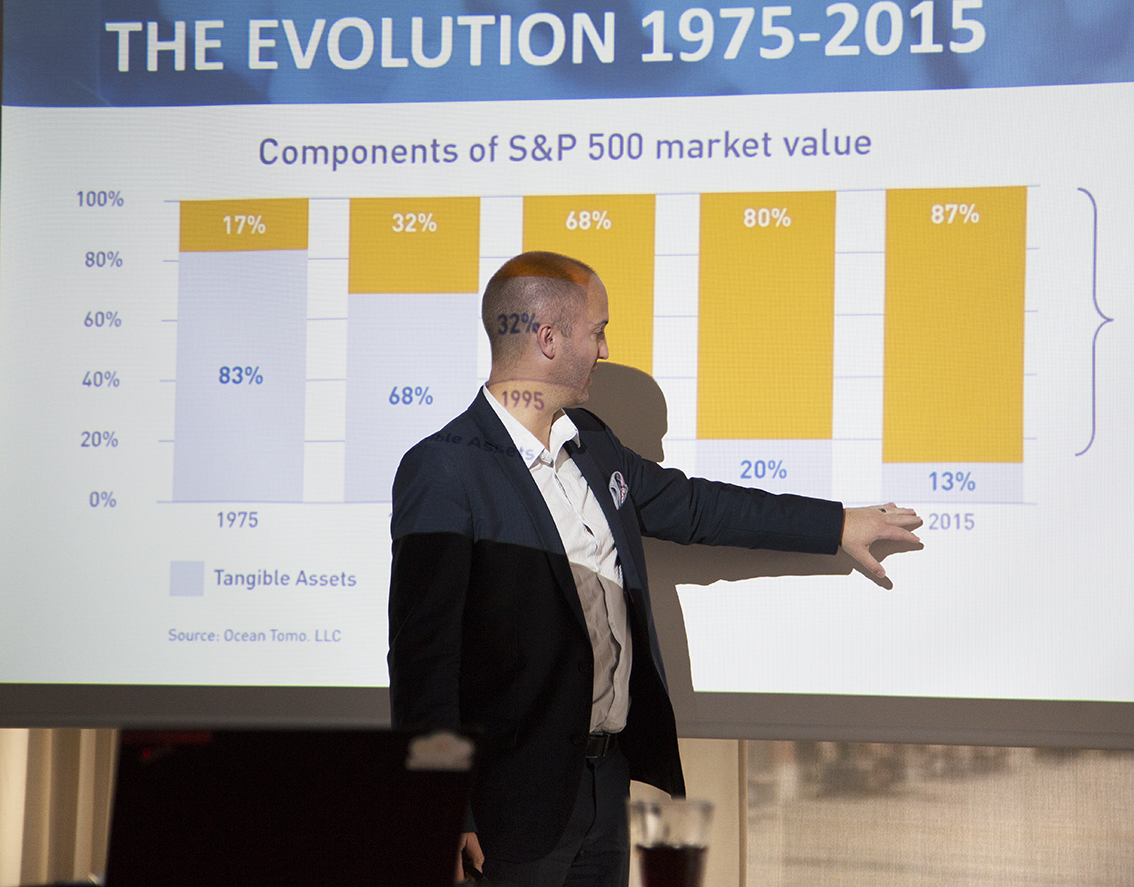The image features a white man with a balding head and short hair, dressed in a dark sport coat and white button-down shirt, standing in front of a brightly lit projection screen. He is pointing at a graph line labeled with the year 2015. The screen's header reads "The Evolution 1975 to 2015" with a subheading "Components of S&P 500 Market Value." A blue banner with white text is displayed at the top of the screen. The left column lists percentages from 100% at the top to 0% at the bottom. Multiple vertical bar graphs, featuring yellow and white colors, represent various statistics over the years. Notably, one bar shows tangible assets at 83% for the year 1975. The source of the data, oceantomo.llc, is noted at the bottom left of the graph. The overall scene is well-lit, highlighting the detailed content of the presentation.